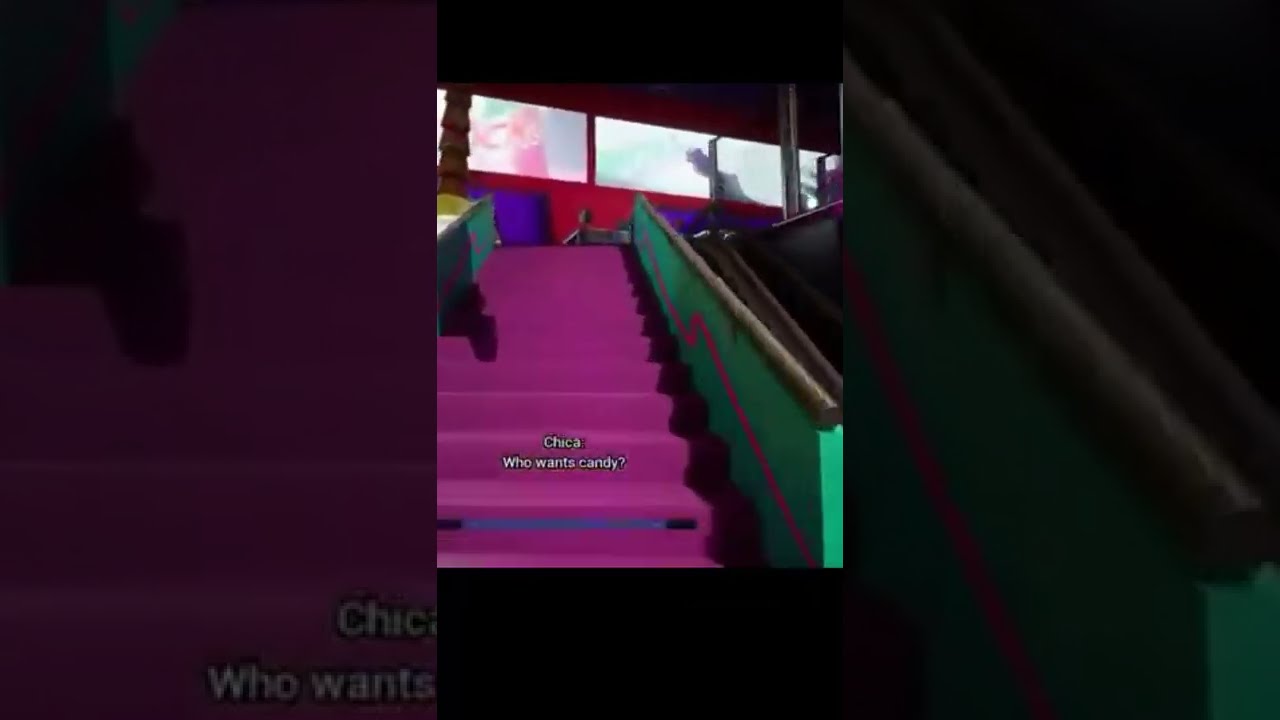The image showcases a vividly colorful staircase with a distinct 80s aesthetic. The staircase itself is painted a bright purple, while the walls flanking it are a vibrant green with a bold red stripe running through them. Extending further upward, the upper walls are painted a striking red, adorned with some photos or images, though they appear somewhat blurred and hard to identify. On the left-hand side, the handrail features yellow detailing. Center stage in this colorful scene is text at the bottom that reads "CHAC3, who wants candy?" This phrase appears twice, adding an element of playful repetition. The upper part of the image is further highlighted by three rectangular sections resembling large video screens or windows. Two of these sections emit a bright white light, obscuring their contents, while the third shows what seems to be a large figure, possibly a poster, looking through. All these elements together suggest that the scene might be from a cartoon or TV show, with its exaggerated colors and animated style.